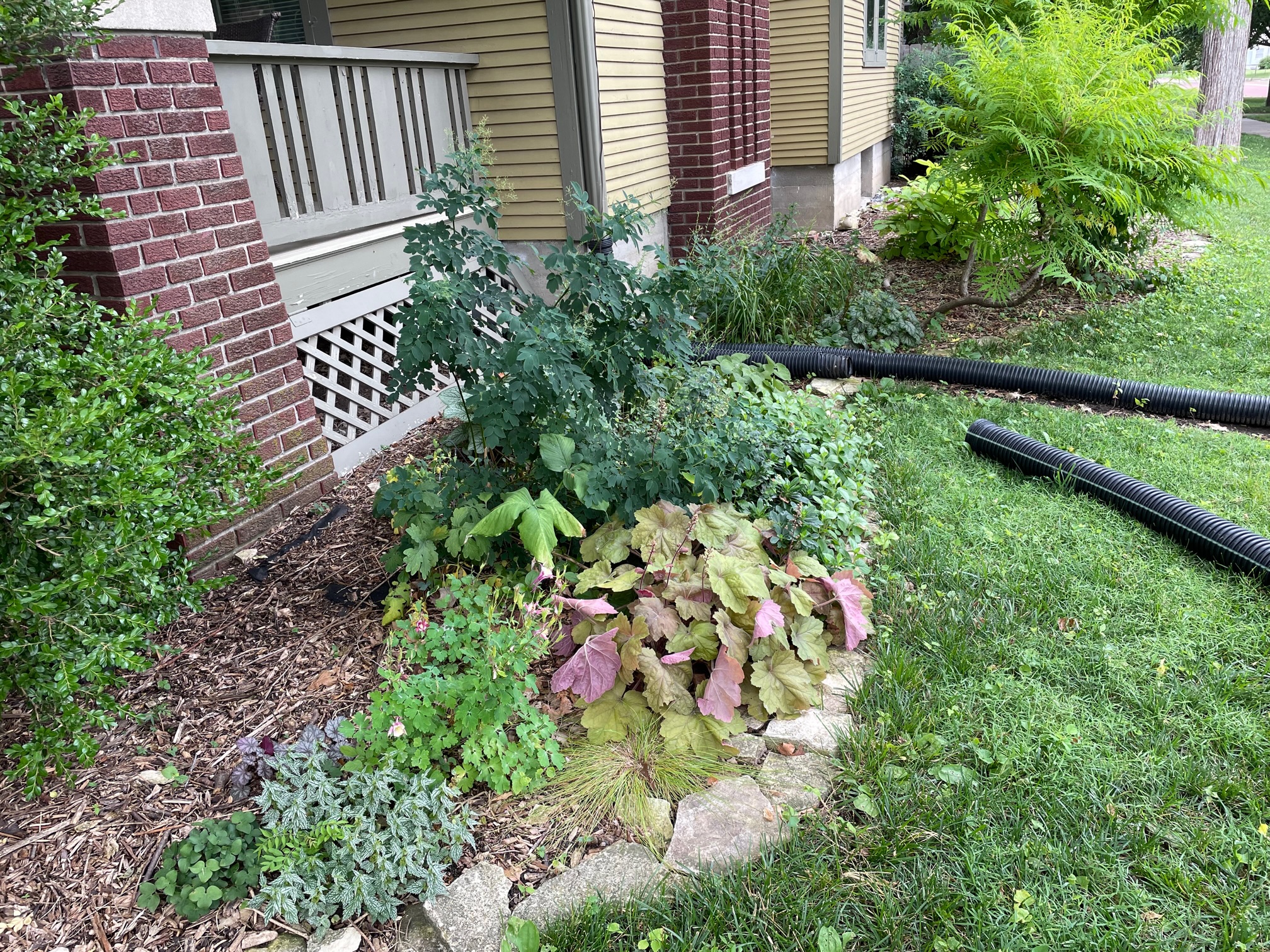This color photograph, taken during the daytime, showcases a detailed section of someone's porch area with a focus on the adjacent garden and flower beds. The porch, made of deep red burgundy brick, features a gray-painted railing and lattice underneath. The house is adorned with tan yellow vinyl siding. The garden includes a variety of plants in a curved flower bed, bordered by rocks and filled with brown mulch. The plant leaves exhibit a range of greens, from sagey to deep forest green, with some having light green with pink undersides. Scattered throughout the scene are black, ribbed downspout extenders and a drain hose, one section of which appears cut and laid out as if about to be positioned. The garden is interspersed with some bright greenery and flowers, albeit with a few wilted ones having pink and brown petals, indicating they're dying. The overall image conveys a well-kept yet slightly aged residential exterior.